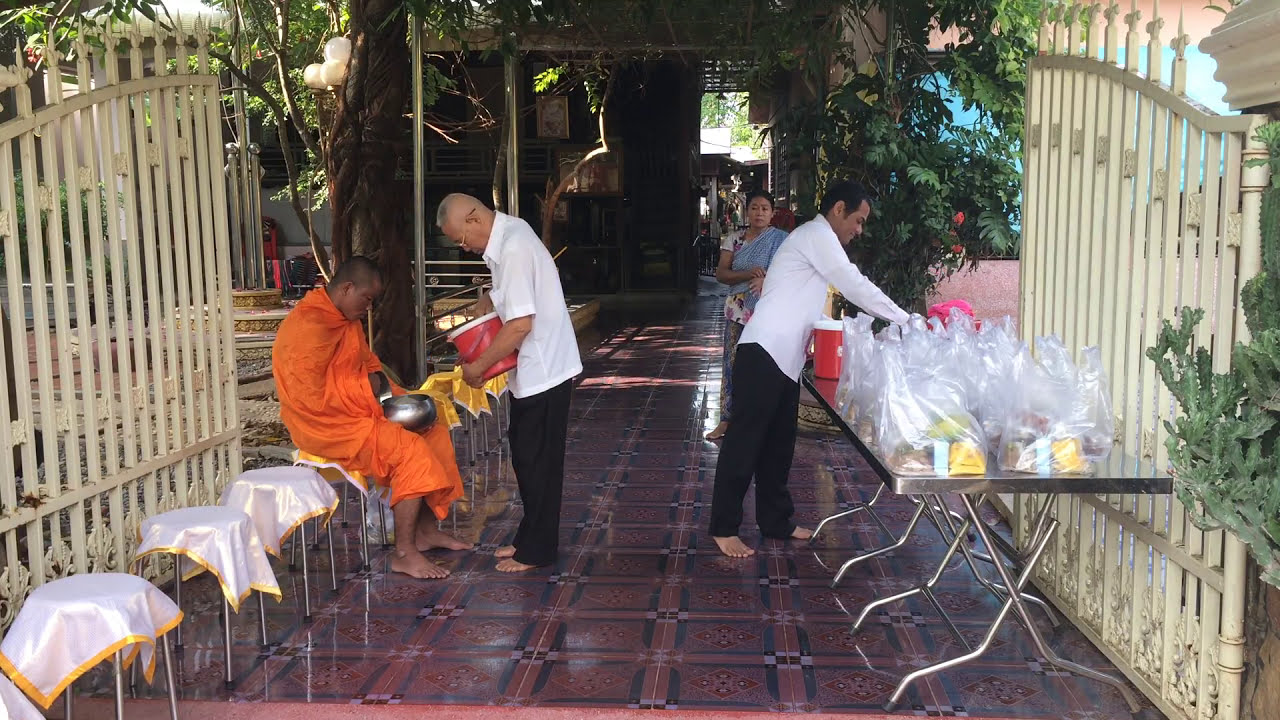The image depicts a semi-outdoor setting, possibly in an Asian country, during the middle of the day. The scene appears to feature a red-tiled walkway leading towards a building entrance, surrounded by white metal gates. To the right of the walkway, there is a table laden with several plastic-wrapped packages, where a barefoot man in a white coat and black pants is tending to the items. On the left side, several stools draped with white cloths edged in gold are arranged, with an individual dressed in an orange robe, perhaps a monk, seated on one of them. The monk is holding a silver object and is interacting with another barefoot man in a white coat and black pants, who seems to be pouring something from a red jug. Both men in white and black are positioned closest to the center of the image. In the distance, a woman in a blue shirt stands facing the walkway, and trees and buildings are visible further off. The overall color palette includes shades of yellow, white, orange, black, brown, tan, green, and red, contributing to the vibrant and detailed atmosphere.